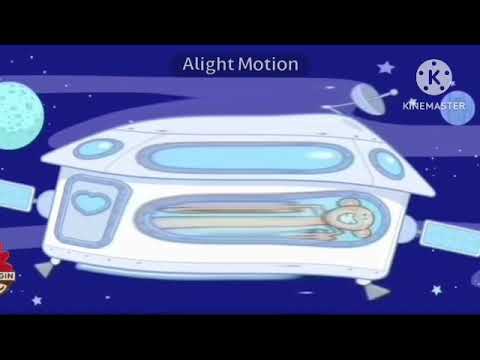The image is a detailed cartoon drawing of a pink spaceship resembling a UFO, floating through space. The spaceship has a distinctive mushroom-shaped top with two blue circular windows on either side and a long rectangular window in the middle. Below these windows, there's another window through which a monkey can be seen inside the spacecraft. An antenna is perched on the right side of the spaceship's top. The background of the image depicts outer space, featuring a blue planet on the left side and several stars. There's also a moon visible in the left corner. The entire scene has a black border on the top and bottom. The text "Alight Motion" is displayed at the back of the image, while "KineMaster" with a 'K' logo is situated in the top right corner. The colors in the image include shades of black, white, gray, blue, purple, light blue, red, and orange. The style is artistic and cartoony.